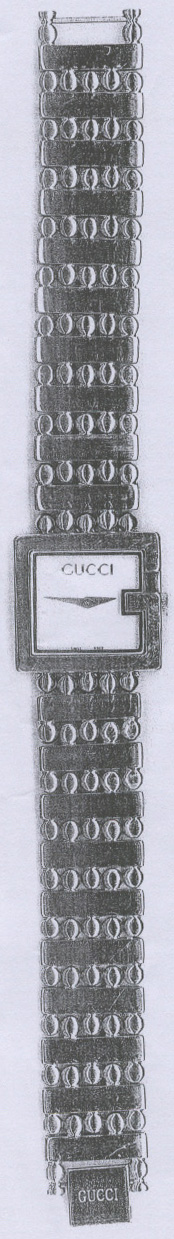The image showcases a luxurious Gucci wristwatch laid out vertically, with its band fully extended from top to bottom. The watch's face, which is distinctly square, prominently features a sleek metallic frame. The pristine white face of the watch lacks any numerical markers or lines, offering a minimalist design. At the top of the watch face, the word "Gucci" is elegantly printed in a thin black font, emphasizing the brand's sophisticated style. The watch hands, indicating the time as approximately a quarter to three, are simplistic yet stylish. Visible at the lower part of the image is the fastening clasp, intricately engraved with the iconic Gucci logo, adding a subtle touch of refinement to the overall design.